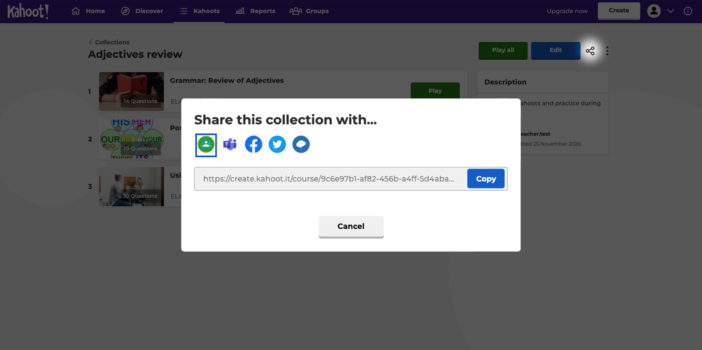The image displays a grayed-out Kahoot website, which appeared after the user clicked the share button. The top navigation bar features several difficult-to-read buttons, likely labeled Home, Explore, and Create. The user's profile icon and name are visible, indicating they are signed in. Below the navigation, there's a section titled "Adjectives Review," part of a grammar collection. Options to play, edit, or share the collection are also present. The prominent share pop-up is a white rectangle labeled "Share this collection with,” offering sharing options via Facebook, Twitter, and an unnamed messaging platform. It allows users to input the Kahoot number or URL, copy it, and share it, enabling resource sharing among school colleagues.